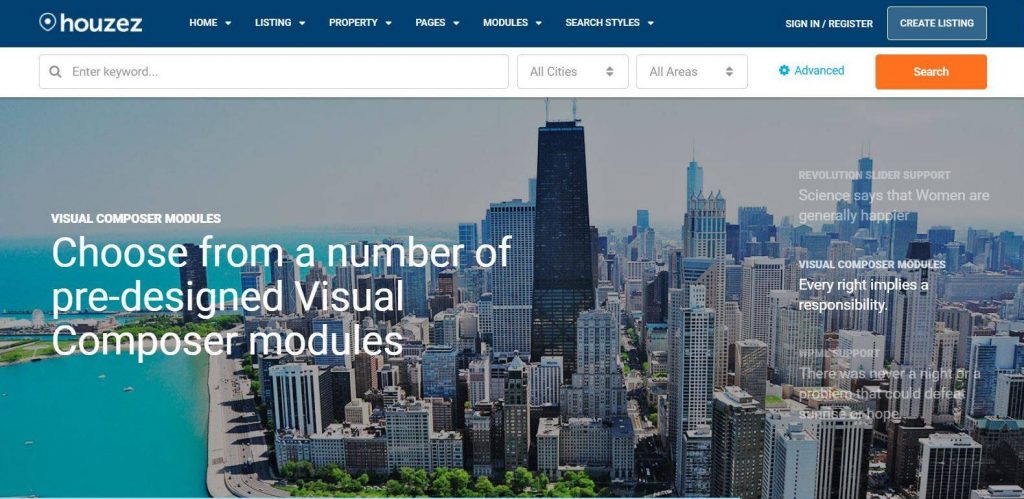This image features a detailed screenshot of the Houses (H-O-U-Z-E-Z) website. The top-left corner prominently displays the brand name "Houzez". The website’s navigation bar includes six categories labeled: Home, Listing, Property, Pages, Modules, and Search Styles. To the right side of the navigation bar, there are options for Sign-In/Register and Create Listing.

Beneath the navigation bar, the interface includes a search section where users can enter keywords, choose from options like All Cities and All Areas, and access advanced search options. The search function is complemented by an orange search button located on the right.

The central portion of the screen showcases a city’s landscape from a high vantage point, depicting a serene body of water to the left and a gray sky above. Overlaid on this backdrop, the left section features the text "Visual Composer Modules" in small white font followed by a larger caption, "Choose from a number of pre-designed Visual Composer Modules".

On the right side, there are three sentences in white text, with the top sentence reading, "Revolution Slider Support Signs says that women are genuinely happier". Below this, it states "Visual Composer Modules, Every Right Implies a Responsibility". At the bottom, faded gray text reads, "there is never a right or a problem that could defeat something hope".

This comprehensive screenshot captures the website’s core elements from the top navigation bar to the detailed search tools and the visually appealing cityscape.